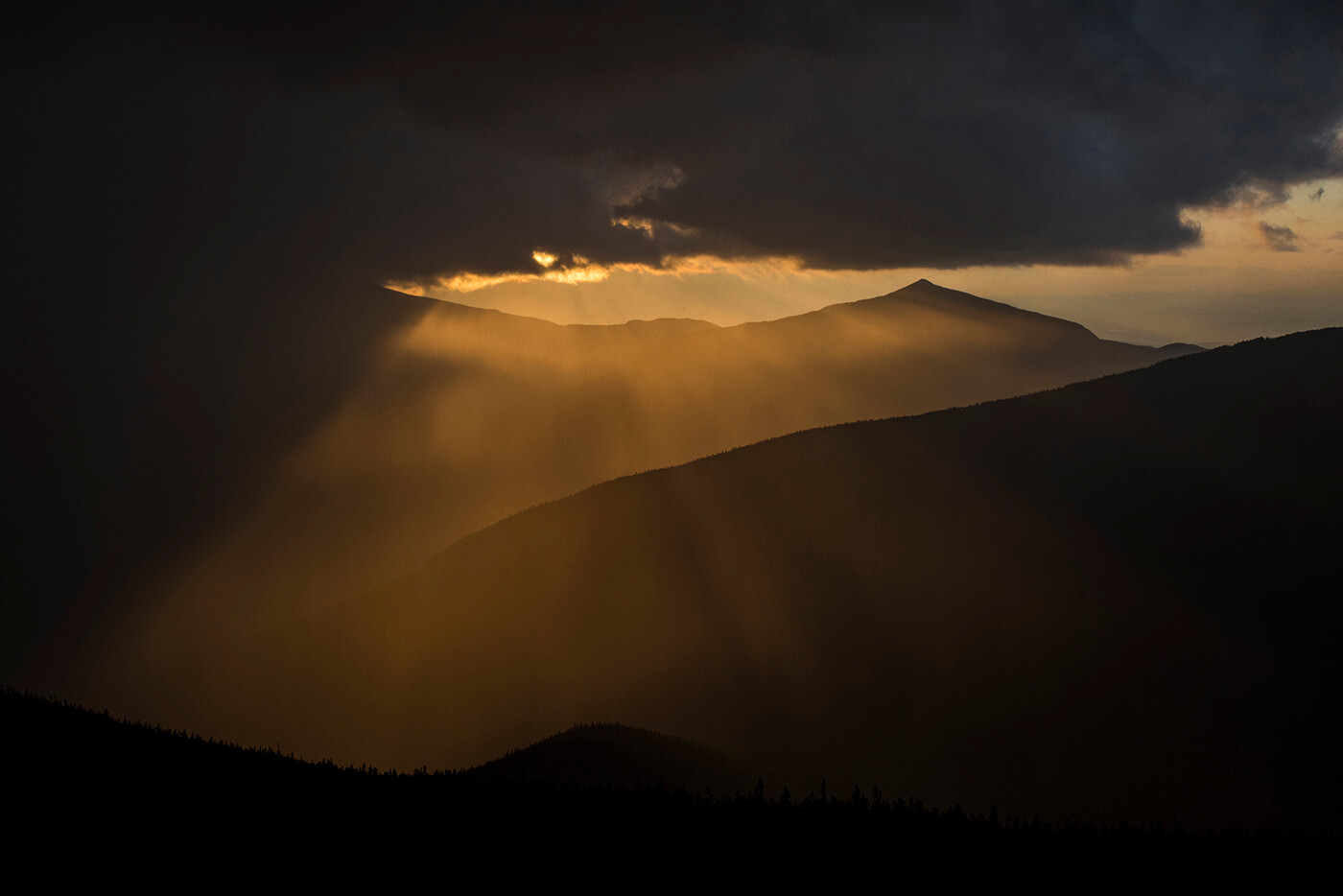This image, whether a hyper-realistic painting or a whimsical photograph, captures an ethereal moment of either sunrise or sunset. The sky is dominated by a mass of very dark grayish-blue clouds, almost as if bruised with shades of blue and purple. These clouds block out much of the sun, yet beneath them, rays of golden and amber light pour through, casting their glow over the landscape. At the forefront, a dark silhouette of hills covered in the tips of pine trees creates a stark black barrier. This is followed by a larger, distant hill occupying the lower right half of the scene, also dotted with pine trees. Beyond this, a range of two towering mountains—one peaking sharply towards the middle right-hand side, the other trailing from the upper left—are bathed in the sun's muted glow. The light, almost magical, caresses the peaks and valleys, rendering them with hints of yellow, gold, and perhaps a touch of orange and peach. This interplay of light and shadow across the mountains and the dramatic sky creates a surreal and captivating visual experience that blurs the line between reality and art.